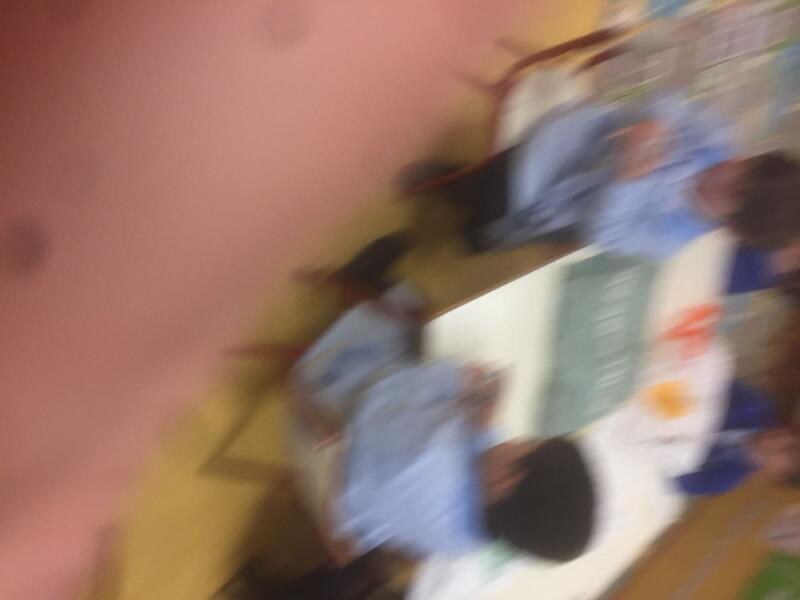This photograph is extremely blurry, making it challenging to discern its contents clearly. The left side of the image features a pinkish salmon hue that appears to be a wall. On the right side, initially, it looks like clutter but upon closer examination from a different angle, it becomes evident that there are two individuals seated in chairs. The photo seems to have been taken upside down, positioning the individuals inversely. Both individuals are dressed identically in blue long-sleeve dress shirts and black pants. They have dark brown hair and sit on red-framed chairs at a white table. On the table, amidst some clutter, a noticeable green piece of paper can be seen. The overall impression suggests this may be an accidental photograph.